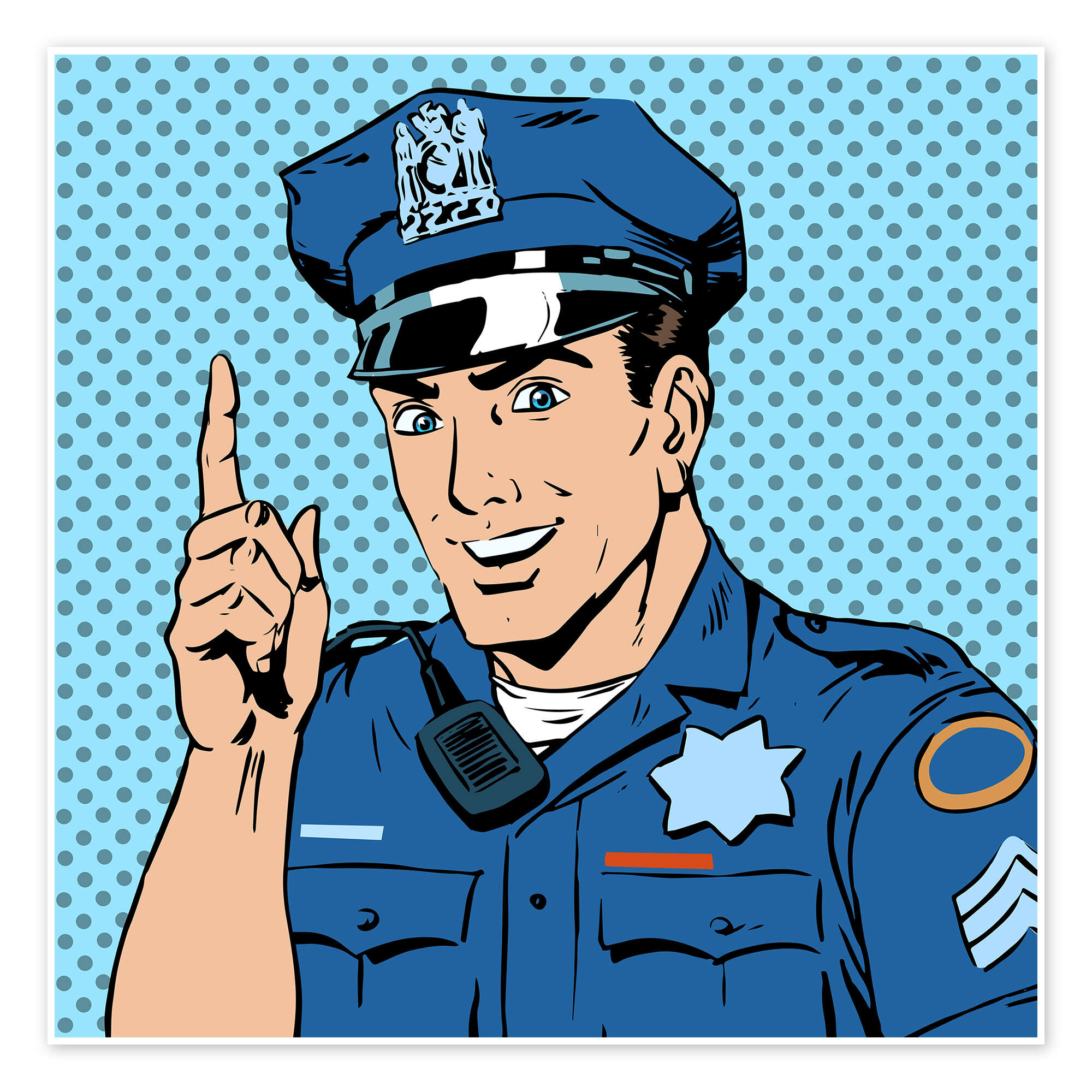The image showcases a detailed comic-style digital illustration of a police officer, depicted from the chest up against a turquoise background adorned with dark bluish-gray polka dots that resemble wallpaper. The officer is dressed in a blue uniform with a distinct star-shaped badge on his chest, a walkie-talkie attached to his shoulder, and an insignia with three upward-pointing arrows on his sleeve. He has light blue eyes and is portrayed smiling, with his right hand (our left) raised and his index finger pointing upwards. The uniform includes an old-style blue police hat featuring a detailed seal with two figures and an animal in between, accompanied by a black visor. A thick white border frames the entire image, accentuated by a thin inner white border that separates the illustration from the patterned background.